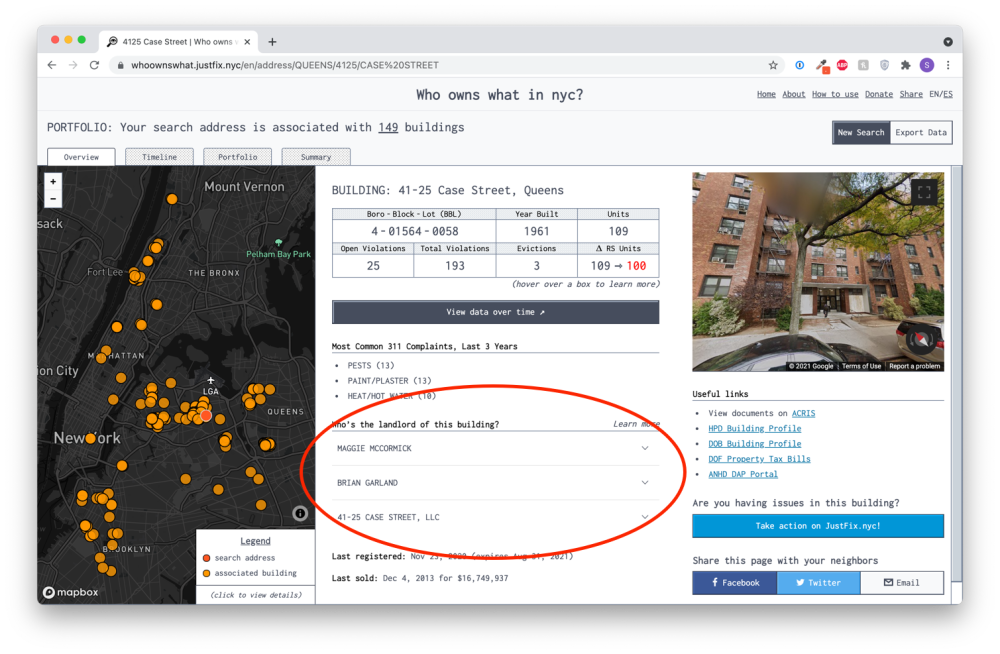This detailed caption describes an image of a web page displaying search results for a property at 41-25 Case Street in Queens, New York:

---

The image shows a web page, likely the result of a property search on the website "whoownswhat.justfix.nyc." At the top, there is a search bar containing the address "4125 Case Street." Above the search bar is the URL: "whoownswhat.justfix.nyc/en/address/queens/4125/Case%20Street." Below the search bar, a header reads "Who Owns What in NYC?" accompanied by several clickable links labeled "Home," "About," "How to Use," "Donate," and "Share," with language options "EN/ES" on the right.

On the left side of the page, a map with a black background and orange circles is displayed, indicating various data points. Headings above the map include "Overview," "Timeline," and "Portfolio." Central to the page, large text indicates the building's address, "41-25 Case Street, Queens." Beneath this, detailed information about the property is provided, such as the year it was built, number of units, open violations, total violations, evictions, and RS units. An option to "View Data Over Time" is available below this section.

Further down, it lists the most common complaints in the last three years, which include pests, paint/plaster issues, and problems with heat or hot water. A highlighted section, circled in red, answers the question "Who is the landlord of this building?" naming Maggie McCormick and Brian Garland, with the owning entity listed as "4125 Case Street LLC."

To the right of the central information, there is an image, presumably of the apartment building in question. This image seems to be sourced from Google Street View as indicated by the markings "2021 Google," along with "Terms of Use" and "Report a problem."

Below the image, there are several useful links, including options to view documents on various platforms: "ACRIS," "HPD Building Profile," "DO6 Building Profile," "DDF Property Tax Bills," and the "HDDAP Portal."

---